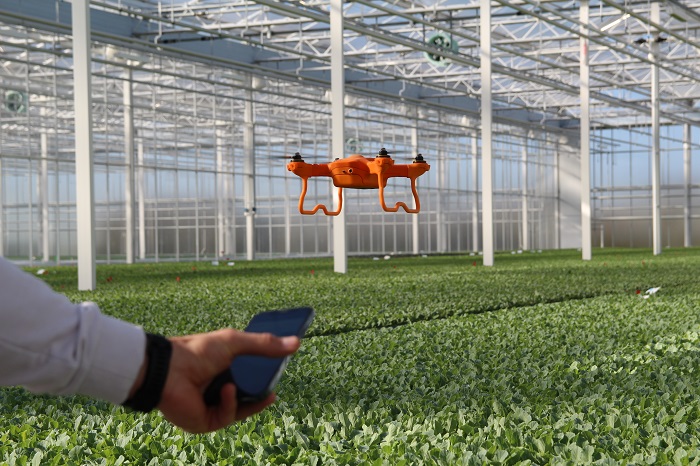A man, possibly a scientist, is controlling an orange drone with his black-cased iPhone in a greenhouse. He wears a white long-sleeved shirt over a black shirt and has a black wristwatch on his left wrist. The drone, equipped with four black propellers and wire-shaped landing gears, hovers over a field of short green leafy plants, possibly spinach. The greenhouse features tall white columns supporting a metal framework and a glass ceiling, with large glass panels on the walls crisscrossed by white bars. There's a plastic sheet visible, separating this field from another on the left.